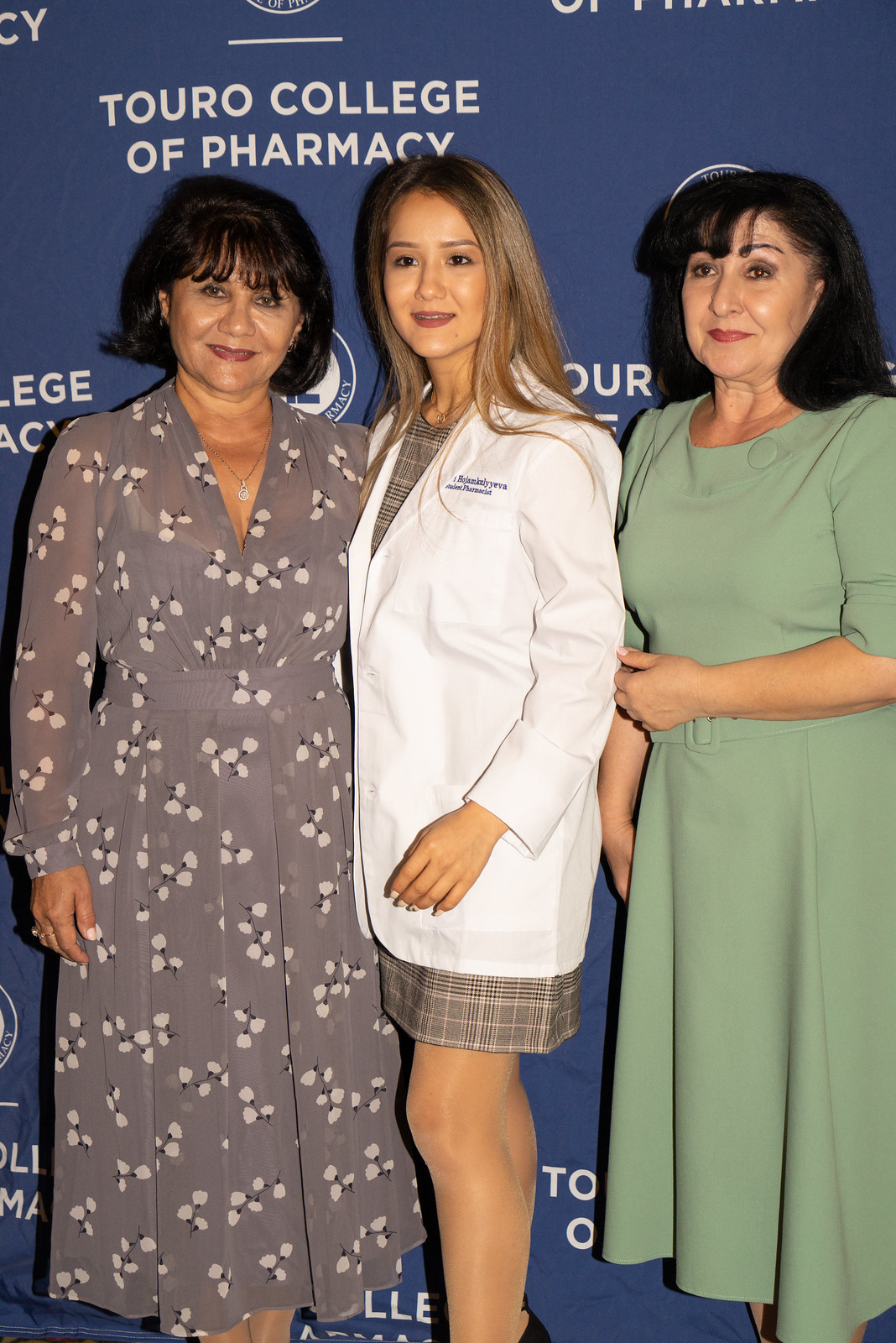The image depicts a vivid, celebratory moment featuring three women posed in front of a dark blue wall emblazoned with the text "Touro College of Pharmacy," suggesting a graduation or a professional event. In the center stands a young Asian woman, presumably a pharmacy graduate, clad in a white lab coat with her name embroidered above her left breast, and a dress beneath that extends just above her knees. Her long brown hair cascades past her shoulders, and her expression is directed towards her left, revealing her youthful and tanned complexion.

To her left is an older woman, possibly in her 50s, dressed in a distinguishable long gray dress adorned with semi-see-through sheer material and white floral patterns. She has shoulder-length black hair, soft tan skin, and bangs. On her right stands another older woman wearing a light green dress with half sleeves. She, too, has long black hair with bangs and a slightly fuller figure. The overall composition suggests a family or close-knit trio, united in celebration, with the older women possibly being her mother and aunt, or sisters, adding to the familial warmth of the moment.